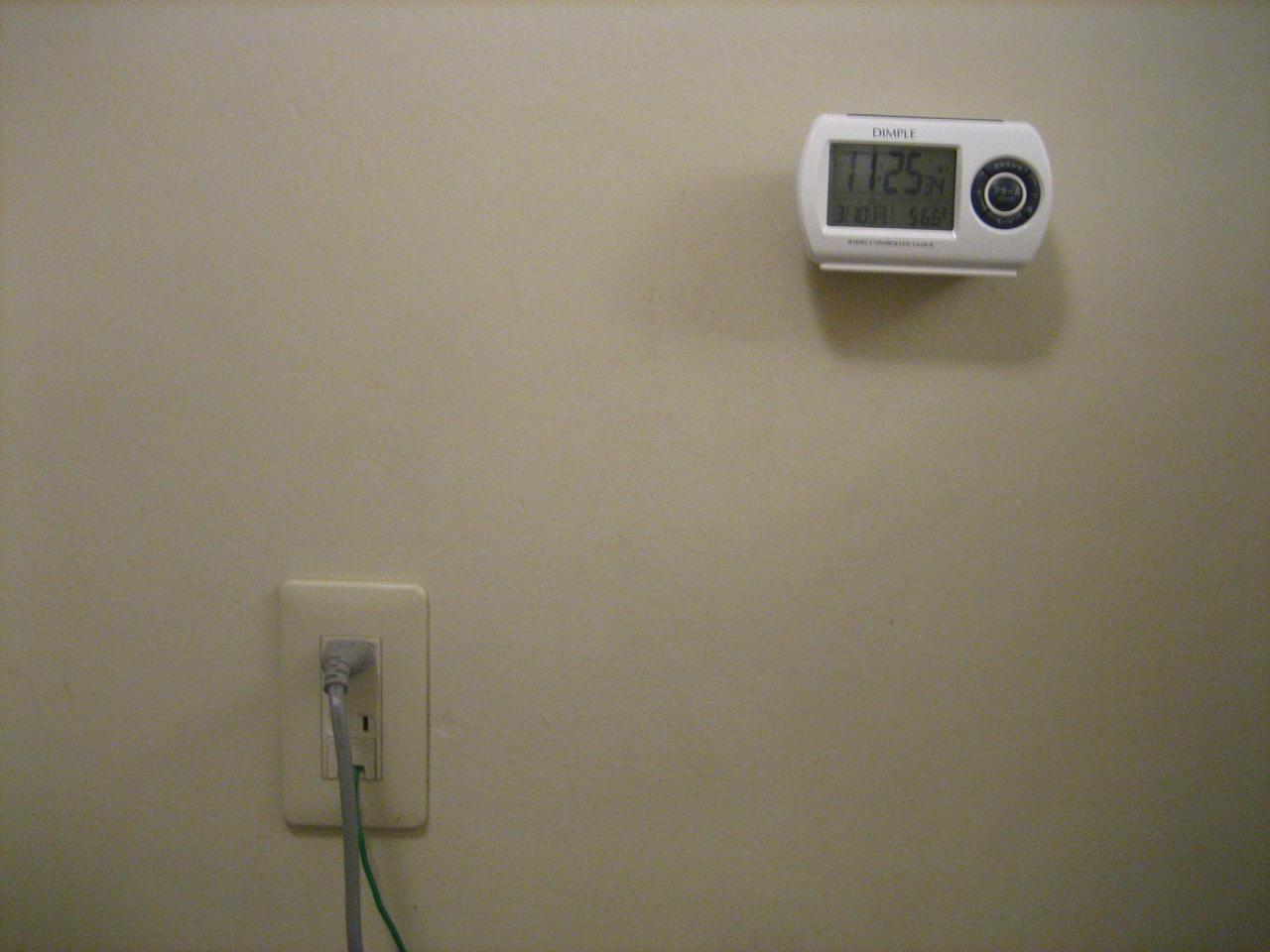In this image, there is a device mounted on a wall referred to as "Dimple." The device features a digital display showing the time "11:25 and 34 seconds." Additional readings on the display include "566" and "56.6 degrees." Another number displayed is "310." On the right-hand side of the Dimple device, there is a series of buttons arranged in a circular, dial-like formation. The device is housed in a white, box-shaped casing. Also visible in the image is an electrical outlet and a wire, possibly a communications cable, emerging from the wall. This appears to be a product shot focusing on the Dimple device and its surroundings.